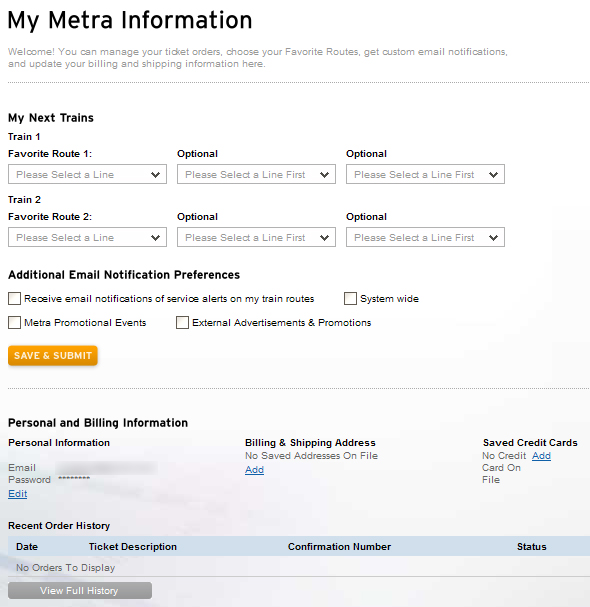This screen capture of a web page is structured into three main sections, each with specific functionalities. The top one-sixth of the page is dominated by the heading "My Metro Information" and a welcome message to the user.

The middle section, occupying about half of the page, begins with the title "My Next Trains." It allows the user to manage their train preferences with several interactive elements. The user can select between different trains and routes using drop-down menus. For Train 1, there are menus for "Favorite Route 1" and two additional options. Similarly, Train 2 has menus for "Favorite Route 2" and two other optional selections. Below this, there's another section titled "Additional Email Notification Preferences," featuring four unchecked checkboxes for "Receive Email Notifications of Service Alerts on My Train Routes," "System-Wide," "Metro Promotional Events," and "External Advertisements and Promotions." A prominent "Save and Submit" button is also present for the user to save their preferences.

The bottom third of the page is dedicated to "Personal and Billing Information." It includes fields for personal details such as email, password, billing and shipping addresses, and saved credit cards, with options to add more information. At the very end of this section, an "Order History" segment lists "Date," "Ticket Description," "Confirmation Number," and "Status." A button labeled "View Full History" provides the option to see a detailed order history.

This effectively structured page ensures users can easily manage their metro information, train preferences, and personal details all in one location.